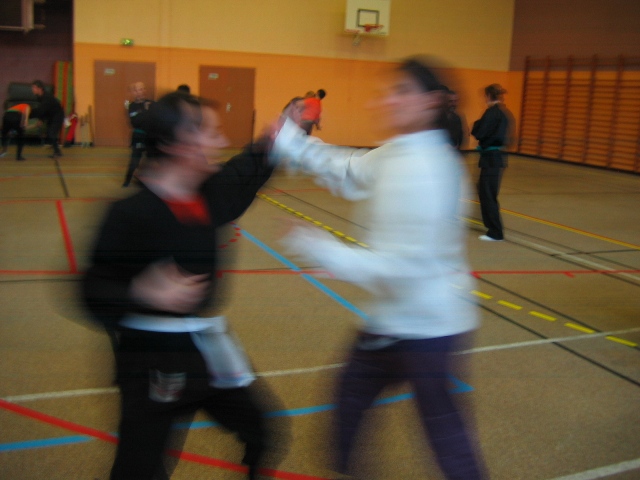This photograph depicts a dynamic scene of a karate class taking place inside a gymnasium with various colored walls, including shades of orange and brown. In the background, a basketball hoop is visible, positioned towards the top side of the image. The gymnasium floor is brown and marked with various colored lines in red, blue, white, and dotted yellow. Near the left-hand side, there are two brown doorways.

In the foreground, the focus is on two women engaged in a fast-paced martial arts exchange, captured in a blurry motion. The woman on the left, dressed in a black karate suit with a white belt, has her left arm outstretched in an attempt to strike her opponent, while her right hand is cocked back, ready for another move. The woman on the right is wearing a white top paired with dark pants. She is blocking the left arm of the woman in black with her right arm, while her left arm appears poised to counterattack.